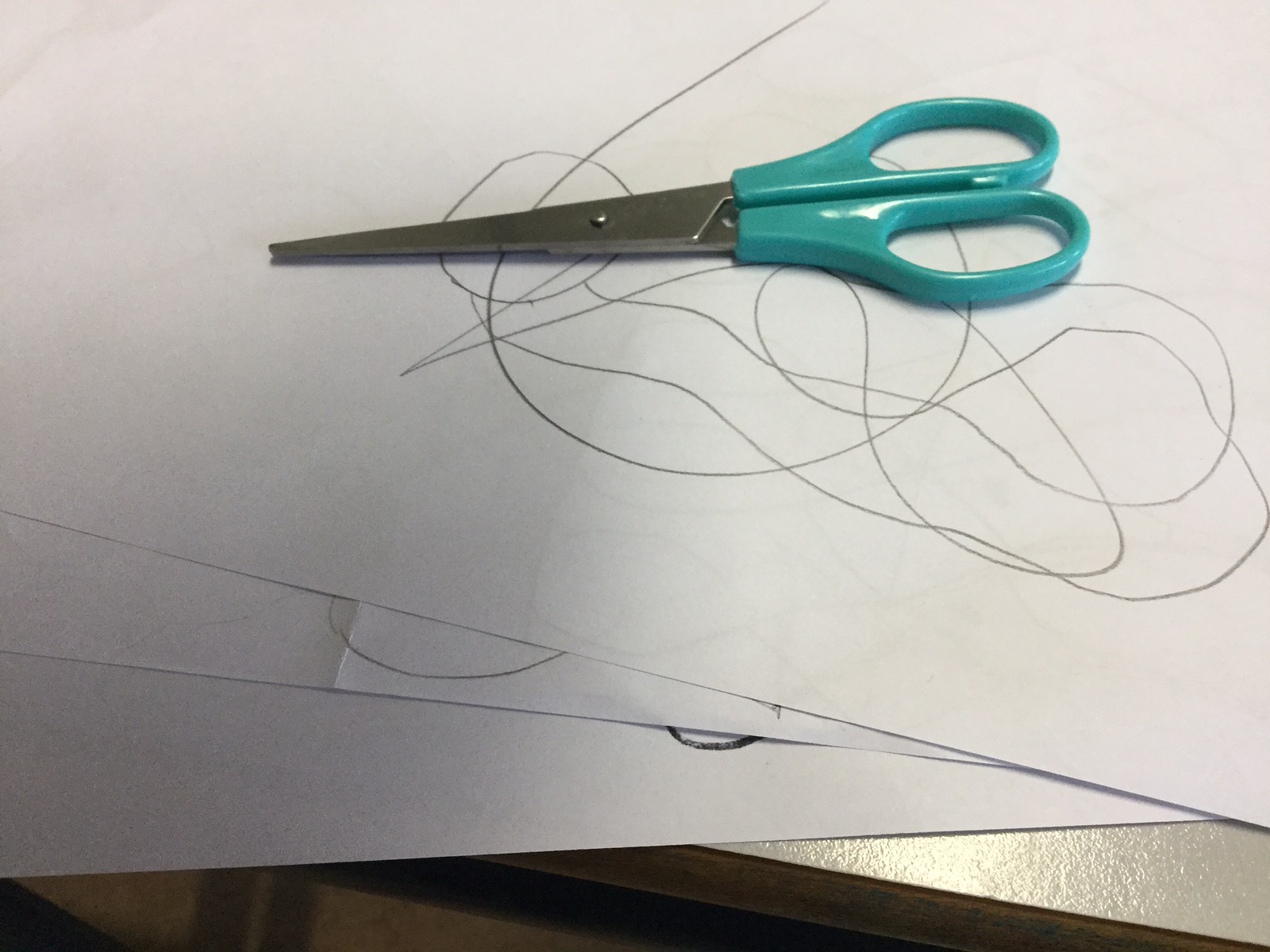This is a detailed close-up photograph featuring a pair of children's scissors with teal seafoam blue handles, lying completely closed on a piece of white paper that has various pencil scribbles and squiggled drawings. The scissors have small, long silver blades, and both the holes for the fingers and thumb are the same size. The paper appears to be part of a larger stack of three layered sheets, with just the upper parts of the underlying papers visible, each having some form of pencil or black arching designs, resembling rows of touching diamonds. This stack of papers is placed on a textured, gray tabletop that has a slightly bumpy yet mostly smooth feel, possibly with a silver hammered metal top and a wood border. The photo also hints at a laminate flooring in the background. The overall scene captures a moment of casual creative activity.